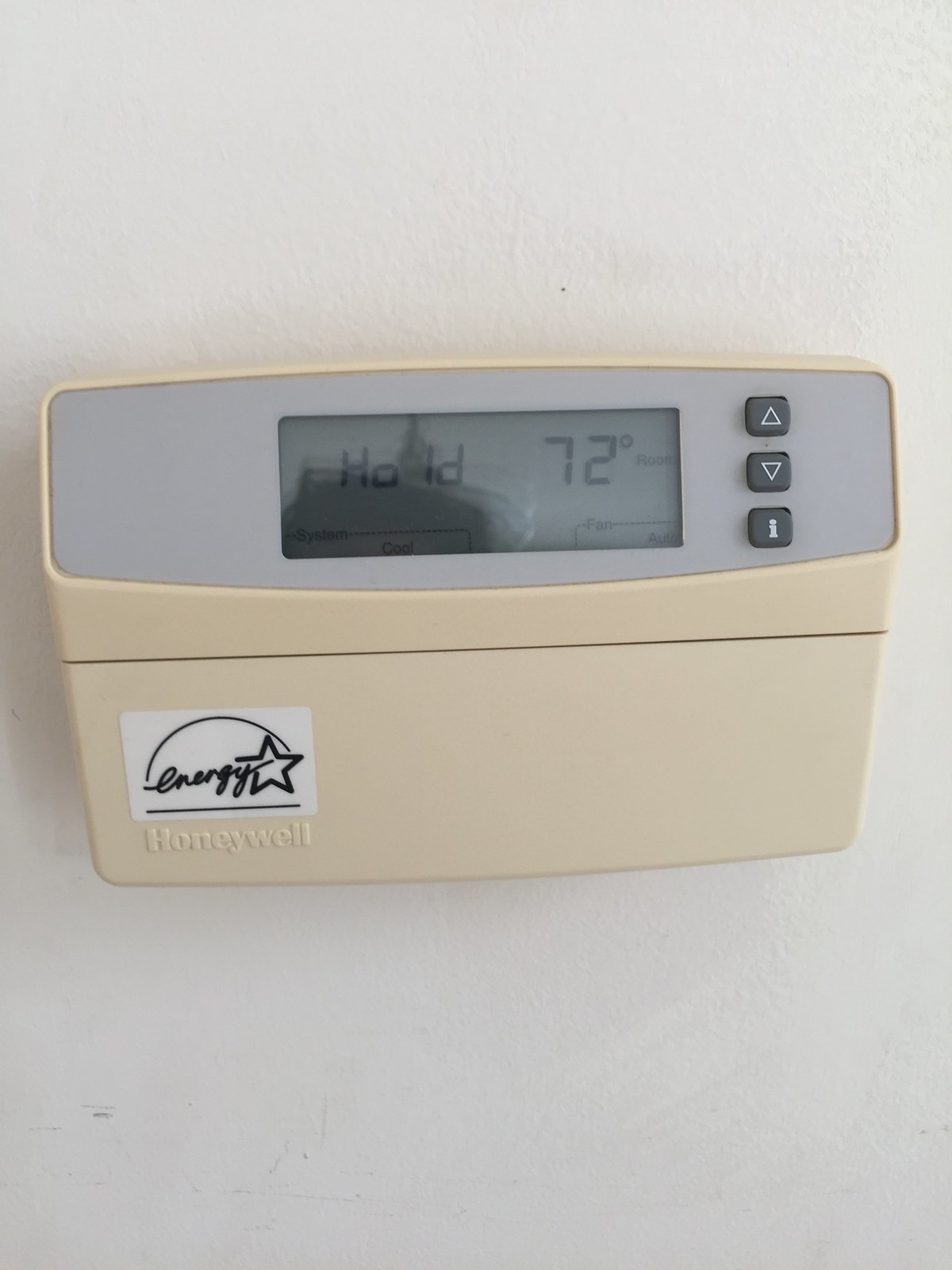The image features a digital thermostat that appears to be quite old, distinguished by its off-white, cream-colored exterior. The thermostat is mounted on a white wall, providing a clear contrast. The central display of the thermostat shows a message: "Hold 72°F," indicating the set temperature. Below this, the display reads "Room" to denote the current room temperature status. In the lower left corner of the screen, the text "System Cool" is visible, specifying that the cooling system is active. In the lower right corner, it states "Fan Auto," indicating the fan mode.

Adjacent to the small screen are three buttons. On the right-hand side, the top button is marked with an upward-facing arrow, which is used to increase the temperature setting. The button below it is marked with a downward-facing arrow, used to decrease the temperature. The third button, located beneath these two, features the letter “I”.

The thermostat also displays the brand name "Honeywell" in the lower left corner, accompanied by the Energy Star certification logo, emphasizing its energy efficiency.